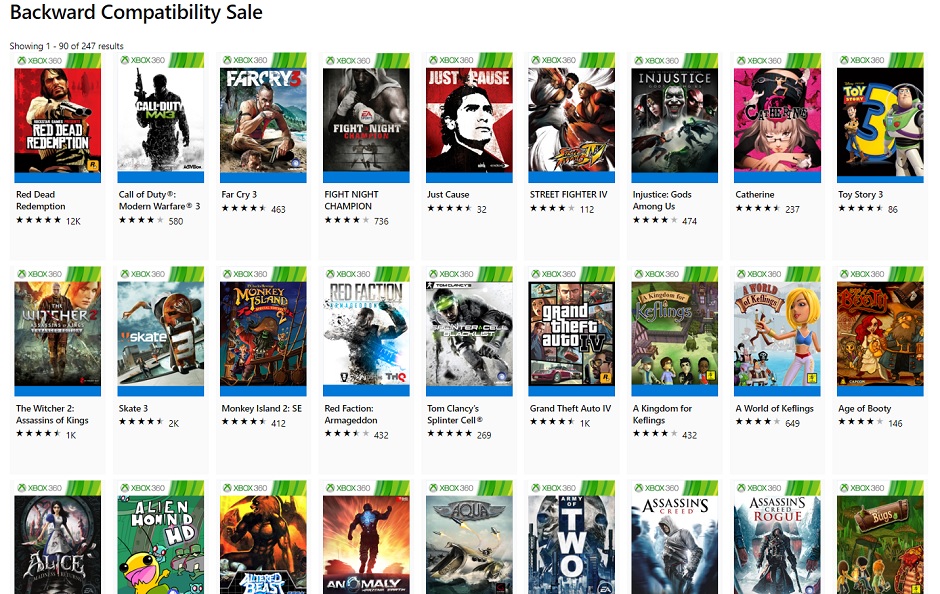"Backward Compatibility Sale"

A promotional banner highlights a "Backward Compatibility Sale" for video games. Viewing options are displayed, indicating "Showing 1 through 90 of 247 results."

**First Row:**
1. *Red Dead Redemption:* Featuring a red background with a man with black hair holding a gun.
2. *Call of Duty: Modern Warfare*
3. *Far Cry:* Depicting a character sitting on a beach.
4. *Fight Night Champion*
5. *Just Cause*
6. *Street Fighter*
7. *Injustice*
8. *Catherine*
9. *Toy Story 3:* Featuring Buzz Lightyear and Woody in the background, with a large yellow number "3" in the center.

**Second Row:**
1. *The Witcher 2*
2. *Skate 3*
3. *Monkey Island*
4. *Red Faction*
5. *Splinter Cell*
6. *Grand Theft Auto*
7. *A Kingdom for Keflings*
8. *A World of Keflings*
9. *Age of Booty*

**Third Row:**
1. *Alice*
2. *Alien Hominid*
3. *Beast*
4. *Anomaly*
5. *Aqua:* Featuring a large mountain in the background with the word "Aqua" above it.
6. *T.W.O.*
7. *Assassin's Creed*
8. *Assassin's Creed Rogue*
9. A game featuring characters standing in front of a green forest (title unspecified).

This detailed list offers gamers a comprehensive view of the diverse gaming titles available during this limited-time sale event.